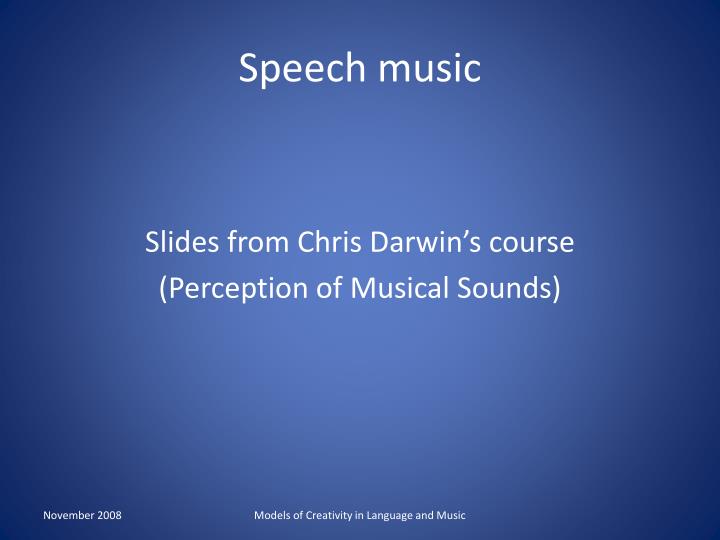The image is a PowerPoint slide predominantly featuring a blue background, which transitions from a darker blue at the edges to a lighter blue in the center. The text is all in white. The largest text at the top center reads "Speech Music." Directly beneath that, in the middle of the slide, is the text "Slides from Chris Darwin's Course," followed by "Perception of Musical Sounds" in parentheses. Near the bottom left corner, it reads "November 2008" in small print. Centered at the bottom of the slide, in similarly small text, is the phrase "Models of Creativity in Language and Music." There are no images or additional elements present, making the focus solely on the textual content.